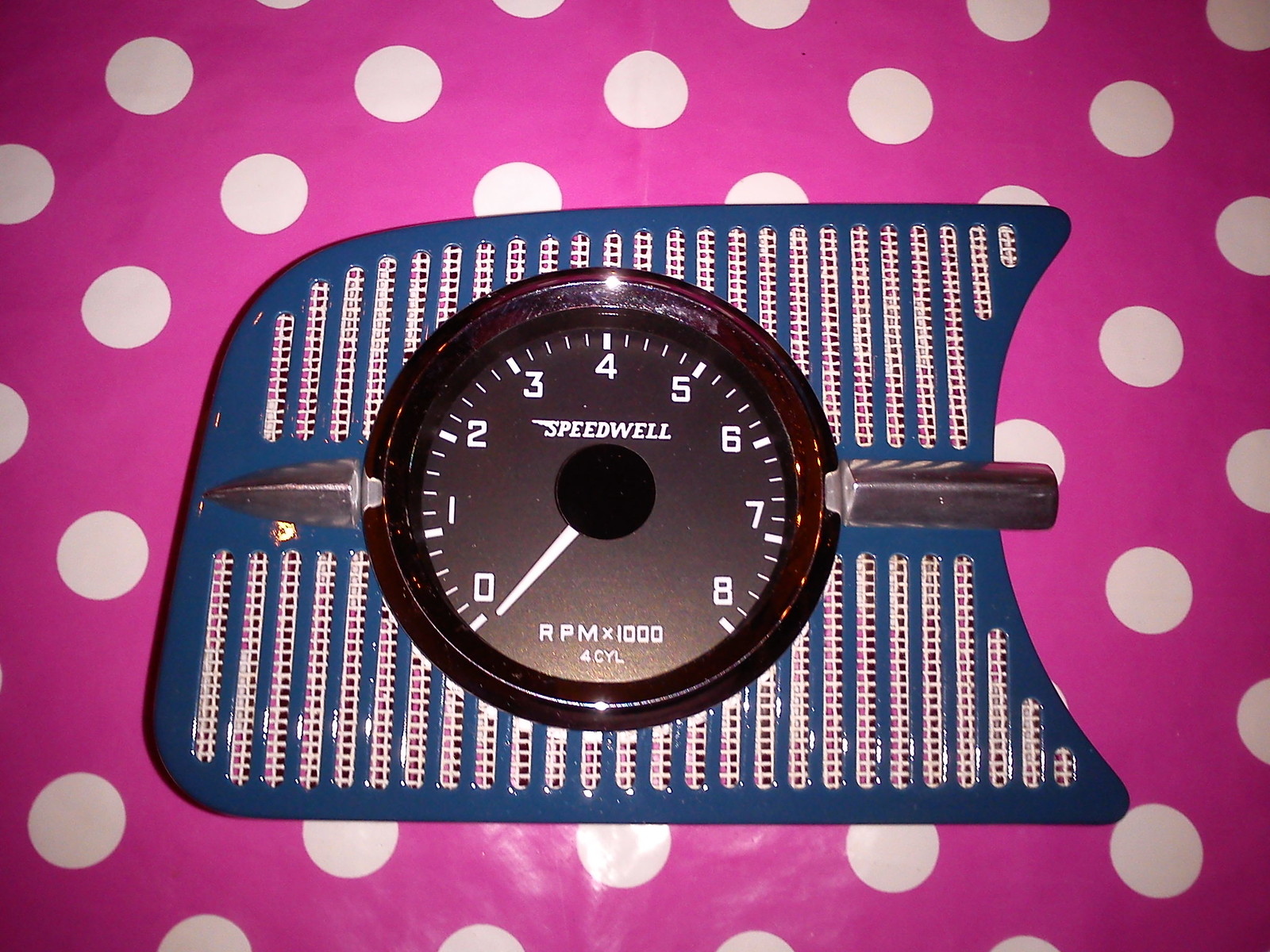The image depicts a unique gauge, resembling a tachometer used to measure RPMs in a car, against a bright pink background adorned with white polka dots. Central to the image is a dark blue, almost rectangular object, featuring vertical stripes of white mesh or netting on its top and bottom. A prominent horizontal metal bar crosses the center, and at the heart of this bar lies a large, round, black gauge. This gauge is marked with white numbers ranging from 0 to 8, indicating RPM multiplied by 1,000. Inscribed within the face of the gauge are the words "SPEED WELL," and at the bottom, it reads "Force Cycle." The gauge's white needle points to zero, capturing a moment of stillness and precision.